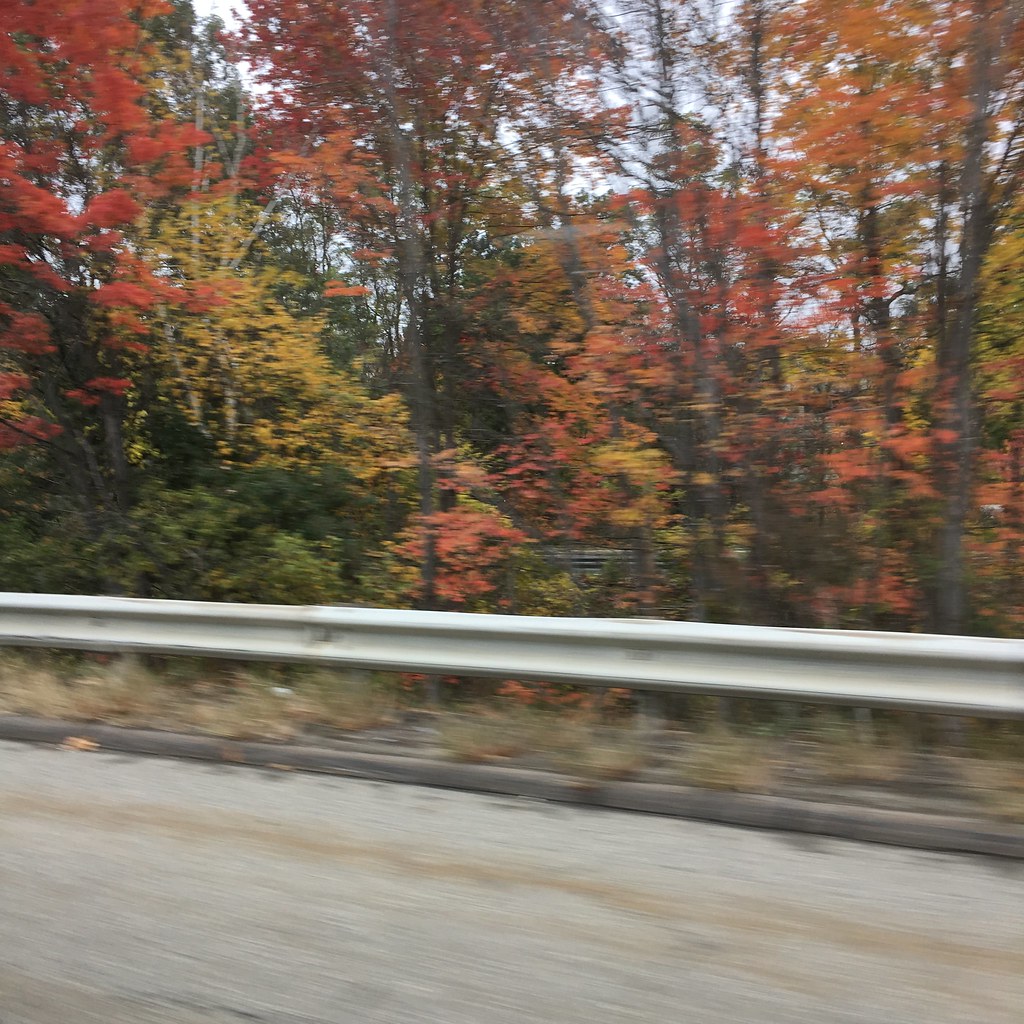The photo captures a roadside scene in the fall, likely taken from the passenger's window of a moving car. In the foreground, a gray concrete curb borders a dark brown road, accompanied by a small grassy area. A light gray, metal guardrail runs horizontally, slightly inclined to the right, serving as a roadside barrier. The background showcases a picturesque autumn landscape with tall trees displaying vibrant fall colors—brilliant reds, yellows, oranges, and patches of green. The sky peeks through the canopy with a grayish hue, adding to the autumnal ambiance. A silver fence with black lines is faintly visible near the base of the trees, contributing to the layered depth of the scene.